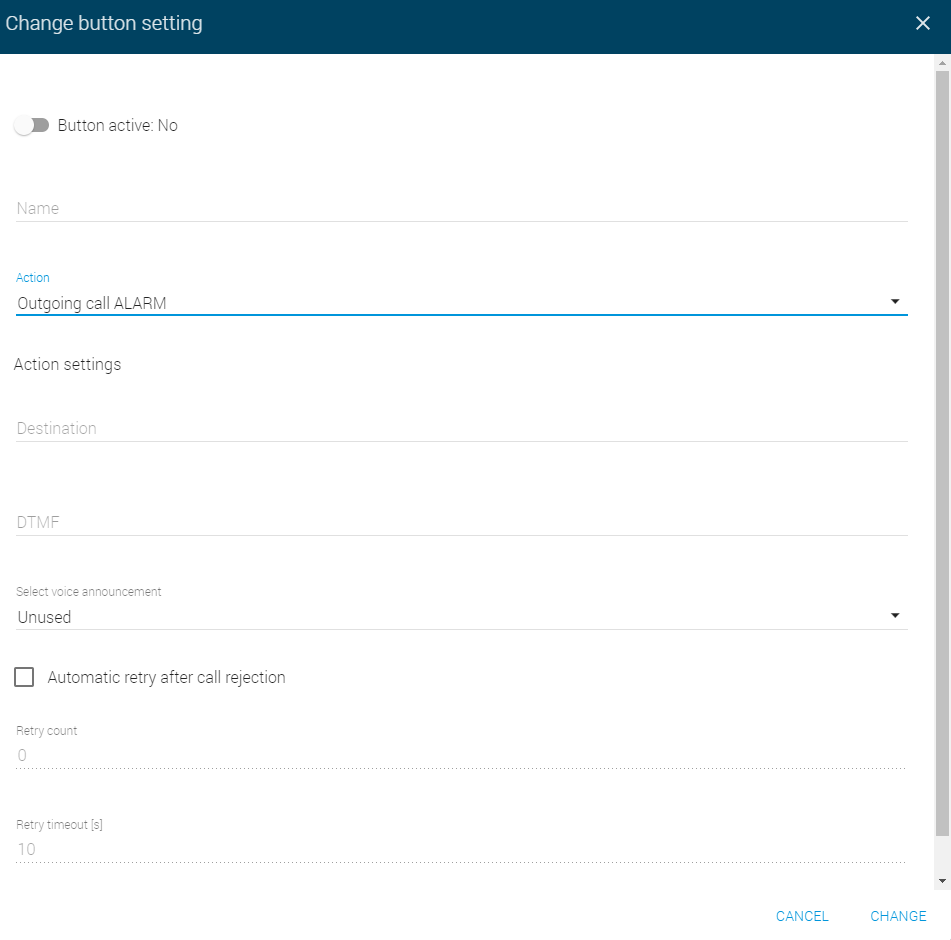This is a cropped screenshot of a website form designed for configuring button settings. The page features a white background with various editable fields and options.

At the top of the page, there is a horizontal bar with a dark blue background and white text that reads "Change Button Setting." Just beneath this bar, there is an option labeled "Button Active" with a toggle switch currently set to "No," allowing users to enable or disable the button.

After that, there is a field labeled "Name" where users can type in their name, accompanied by a dedicated input line. Below this, in blue text, is the label "Action," with a dropdown menu that has "Outgoing Call Alarm" selected — though other actions can be chosen as well.

Following the action section, there is a field under "Action Settings" where users can type in their destination. Another field below this is designated for entering DTMF (Dual-tone Multi-frequency signaling). 

Next, there is an option to select a voice announcement setting, which currently indicates "Unused." Beneath this is an empty checkbox labeled "Automatic Retry After Call Rejection," which users can select if desired.

The section continues with a setting labeled "Retry Count," which is currently set to zero. Following this, there is an option for "Retry Timeout" measured in seconds, showing a current value of 10 seconds.

At the bottom of the form are two clickable options in blue text: "Cancel" and "Change," providing the user with the choice to either cancel their changes or apply them.

Overall, the form allows for detailed customization of button actions and settings, providing multiple editable fields and selectable options for user-specific configurations.